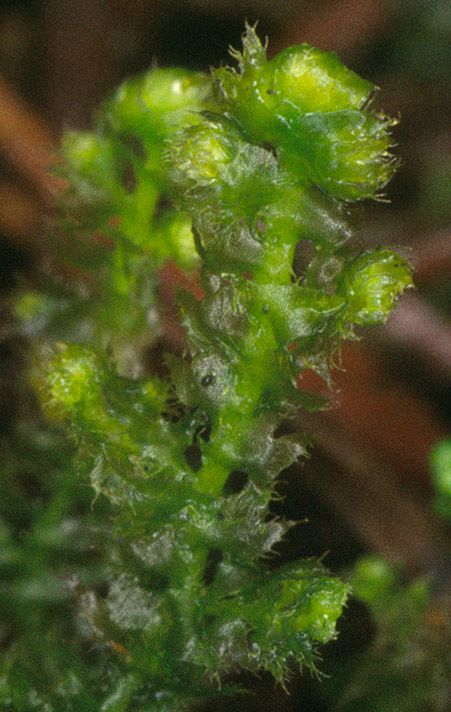This is a close-up photograph of a green plant known as ciliated fringewort (Ptilidium ciliare). The image features a prominent, lime green stem that extends from the bottom left and curves to the right. Along the stem, there are several green buds, darker towards the outside, transitioning to a lime green center with hints of yellow inside. The plant is covered in coarse, fuzzy hairs, giving it a rough texture. The surface of the stem appears shiny, almost like it is covered with a plastic film, possibly due to the lighting. In the blurry background, another similar stem is visible, set against a dark and out-of-focus backdrop, suggesting an outdoor setting, possibly under a pine tree. The overall scene is filled with intricate details highlighting the plant's unique and fascinating structure.